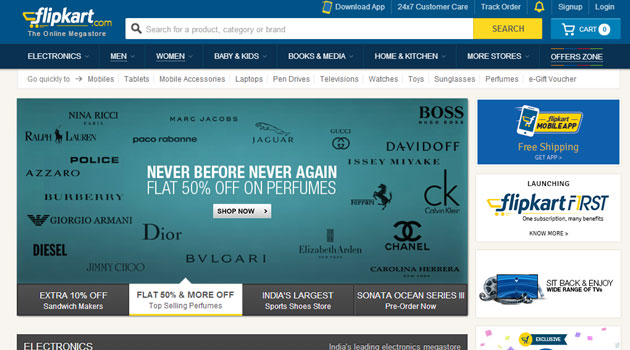This horizontal image captures the homepage of the Flipkart website, viewable on both computers and smart devices. Dominated by a midnight cerulean blue banner at the top, the Flipkart logo appears in white on the upper left corner, accompanied by the text "flipkart.com: The online mega store." To the right, a bright yellow search bar sits beside a blue shopping cart icon that shows zero items.

Above the search bar are several convenient options: a 'Download App' button, 24/7 customer care link, order tracking with a bell icon, and sign-up/log-in options.

Directly below the search bar, a slightly darker navy blue/black menu offers clickable categories, including Electronics, Men, Women, Baby and Kids, Books and Media, Home and Kitchen, More Stores, and Offer Zone. Below this, Quick Links provide faster access to items like mobiles, tablets, mobile accessories, laptops, pen drives, televisions, watches, toys, sunglasses, perfumes, and e-gift vouchers.

The central backdrop features prominent brand names such as Dior, Burberry, Pleece, and Ralph Lauren, promoting a sale with the slogan "Never before, never again: flat 50% off perfumes" and a "Shop Now" button. There's also an option for an additional 10% off and a flat 50% off offer selected. Further promotional content includes details about India's largest sports shoe store and the Sonata Ocean Series. On the right, icons highlight features like free shipping and new launches.